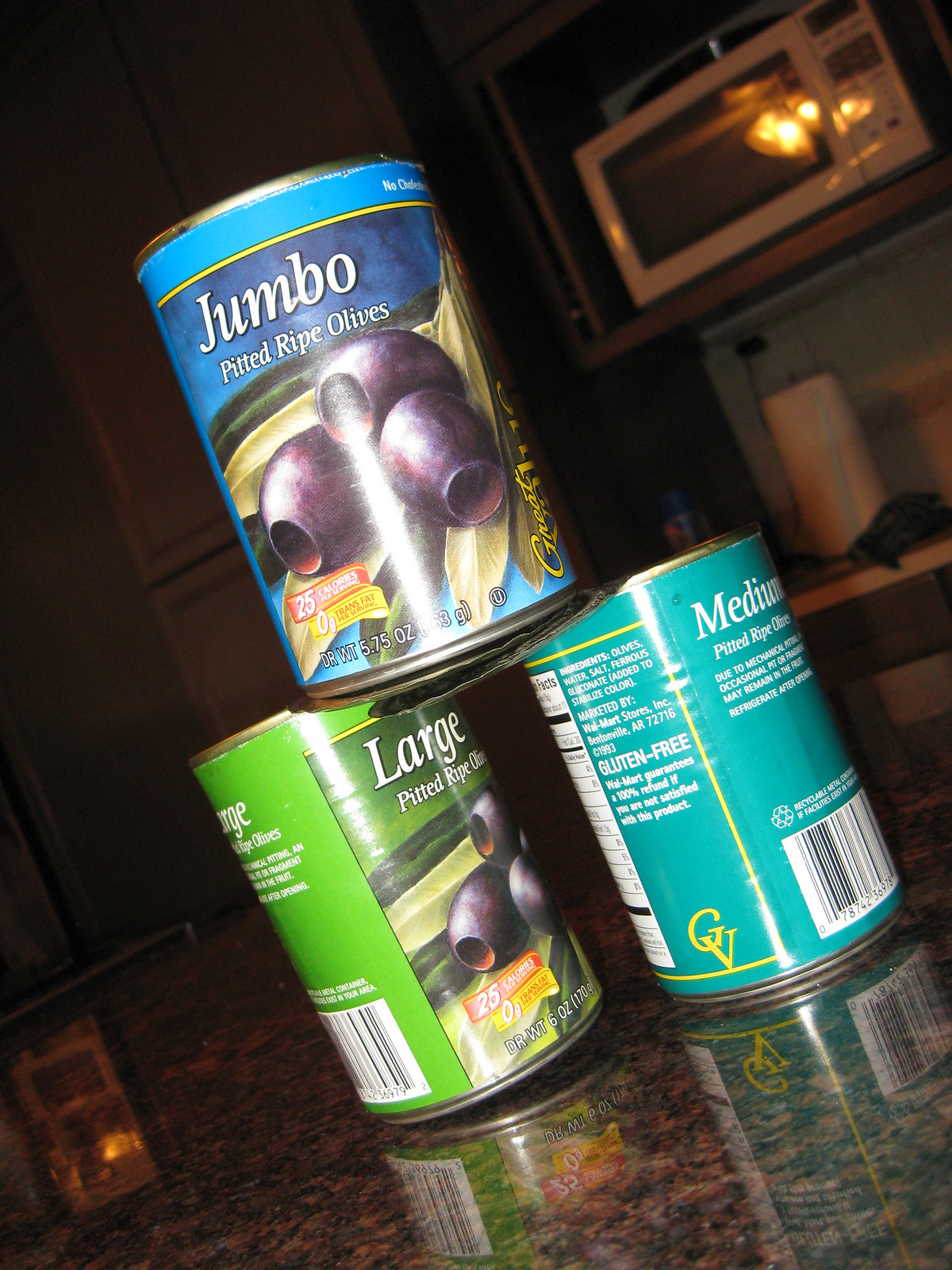This photograph features a trio of aluminum cans, each containing pitted ripe olives, meticulously arranged in a pyramid formation on a sleek kitchen countertop. The can at the apex of the pyramid boasts a blue label, prominently displaying the text "Jumbo Pitted Ripe Olives" along with an illustration of three large black olives. Below it, on the bottom left, is a green can labeled "Large Pitted Ripe Olives," also adorned with an image of three olives, albeit slightly smaller than those on the blue can. Completing the assembly, the bottom right can with a teal wrapper is partially turned, revealing some nutritional information and the text "Medium Pitted Ripe Olives," though the logo image is not fully visible. The well-lit countertop lies in a cozy kitchen setting, with a microwave subtly visible in the background, adding a touch of everyday home ambience to the scene.